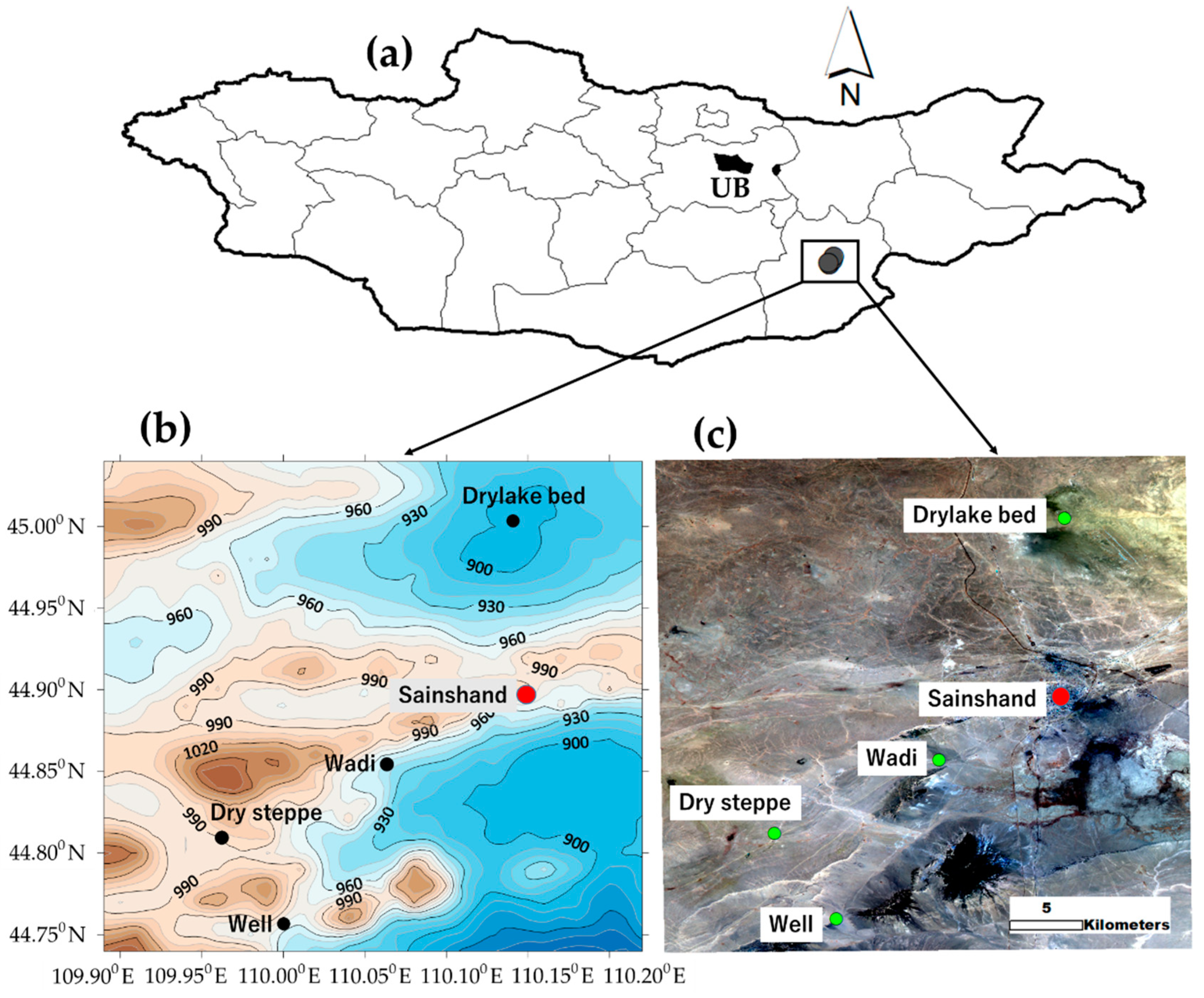This image depicts a detailed composite map labeled with sections A, B, and C. Section A features a black and white graphic of a country or region, delineated by various borders that may represent counties or different administrative divisions. An arrow labeled N points upward, indicating north. To the left of this section, there's text mentioning geographical features like a "Dry Lake Bed," "Seine Shand," "Wadi," and "Dry Step," with a red dot next to "Seine Shand." The scale of this map section is noted to be five kilometers.

Section B presents a more colorful drawn area highlighting land in brown and water in blue. It focuses on the terrain and geographical features more visually, showing islands and bodies of water. Section C, placed adjacent to B, offers a satellite-like image capturing actual terrain details, with clear visuals of the dry lake bed and surrounding landscape. This section also includes latitude and longitude coordinates, with degrees listed on the left side (45° and 44°) and the bottom (109° and 90° E), likely indicating specific locations or alignments on the map. Together, these sections provide a comprehensive overview of a specific region, emphasizing both drawn and satellite perspectives along with detailed geographical descriptions.